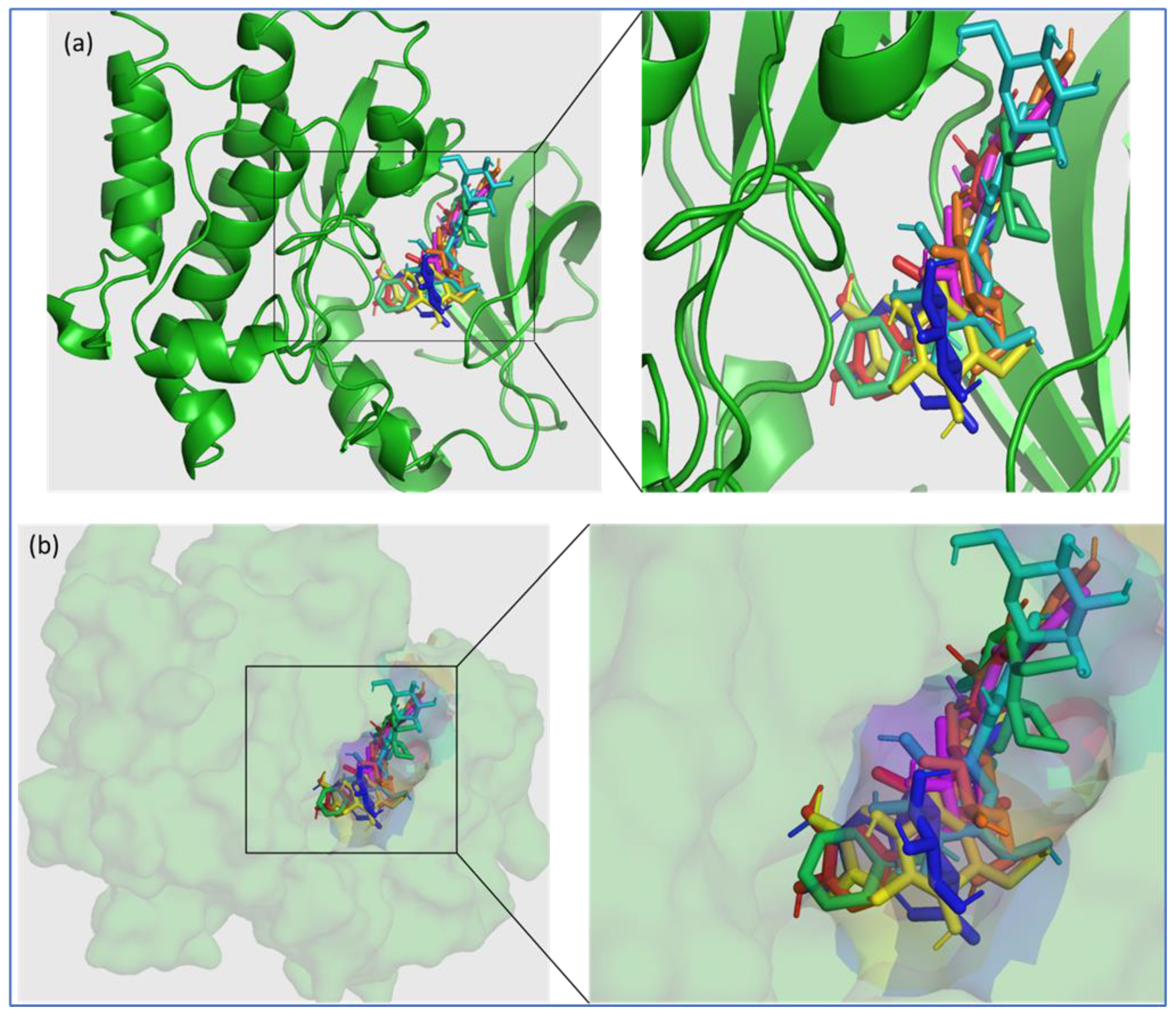The image consists of two panels labeled A and B, each subdivided into four quadrants, set against a gray background. Panel A displays intricate green, ribbon-like structures resembling cellular or protein formations, intertwined with variously colored, smaller ribbon-like structures. The left quadrant of Panel A features a central square connected to the adjacent tile, showcasing larger, brightly-colored ribbon formations akin to DNA strands, densely packed together.

Panel B, positioned below A, emphasizes the DNA-like structures. The right quadrant of Panel B features a close-up view of these structures, revealing a mass of interconnected, multi-colored particles. This close-up appears less sharp and grayish compared to the others, with the DNA-like shapes more prominently displayed. The entire image, with its vibrant animations and complex, curly green forms intertwined with multi-colored ribbon-like elements, suggests a detailed, scientific illustration possibly depicting protein breakdown or cellular structures, minus any accompanying textual descriptions.